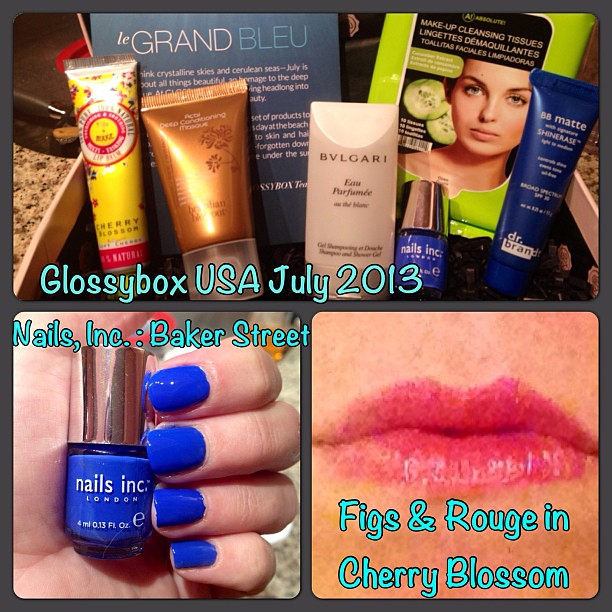This advertisement for women's cosmetics, titled "Grand Blue," features an elegant array of products in a Glossy Box USA from July 2013. The top section of the image showcases an open box containing five distinct cosmetic items, spotlighted against a dark blue placard that reads "Grand Blue." Below, the lower left corner captures a close-up of a woman's hand with nails painted in a vivid blue, holding a bottle of Nails Inc. nail polish in the shade Baker Street. Adjacent to this, the lower right corner presents a close-up of lips adorned with a vibrant pink hue, labeled Figs and Rouge in Cherry Blossom. The photographic composition is a mix of horizontal and square formats, effectively highlighting each product with realism and precision.